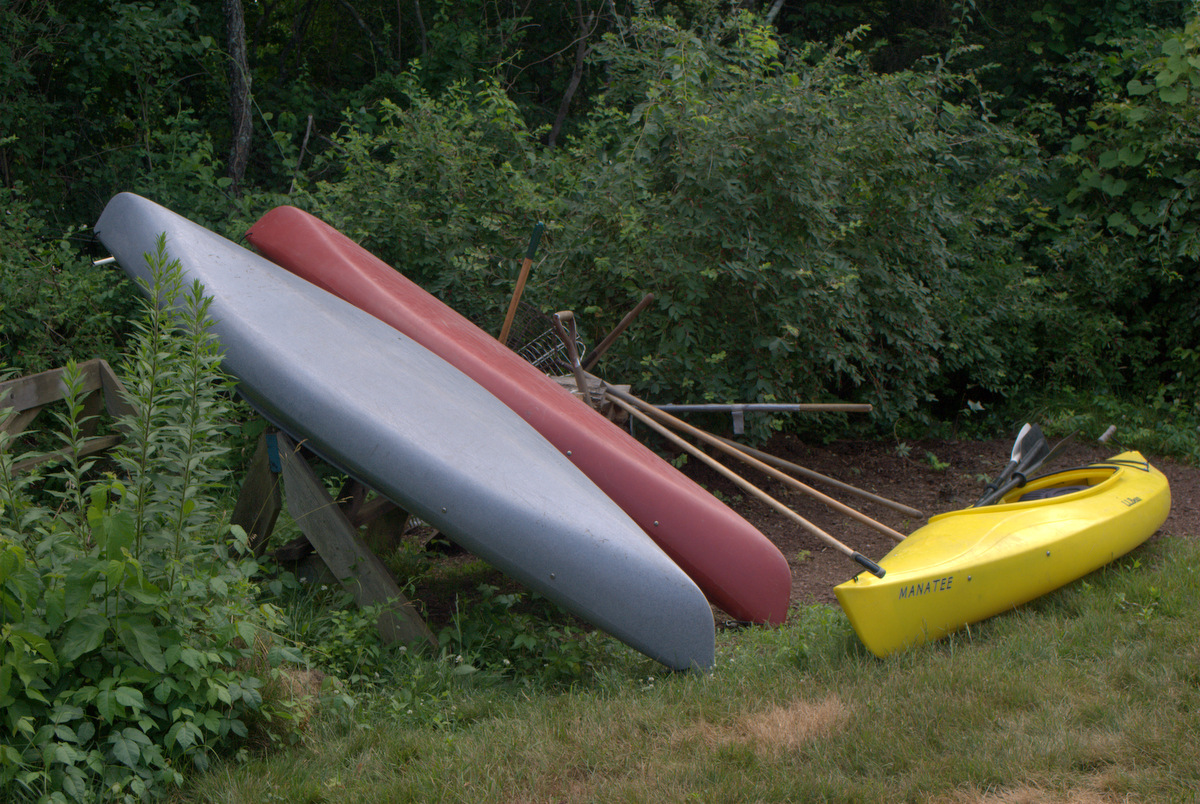This color photograph depicts three people-powered boats arranged on a patchy, green grassy area. A vibrant yellow kayak sits upright on the grass, showcasing the word "Manatee" in black letters on its bow, with its paddles nestled inside the shell. To the left, two more boats—likely kayaks or canoes—are seen leaning upside down against an elevated wooden rack, which appears to be a sawhorse. One of these is a faded red color, while the other is a bluish-gray. Behind the kayaks, a stack of garden tools with long handles, including a pitchfork or hay rake, is visible. The background features a dense forest of deciduous trees and bushes. The foreground is comprised of short grass dotted with tall weeds, especially on the left side near the canoe rack, and a patch of exposed dirt can be seen next to the yellow kayak.